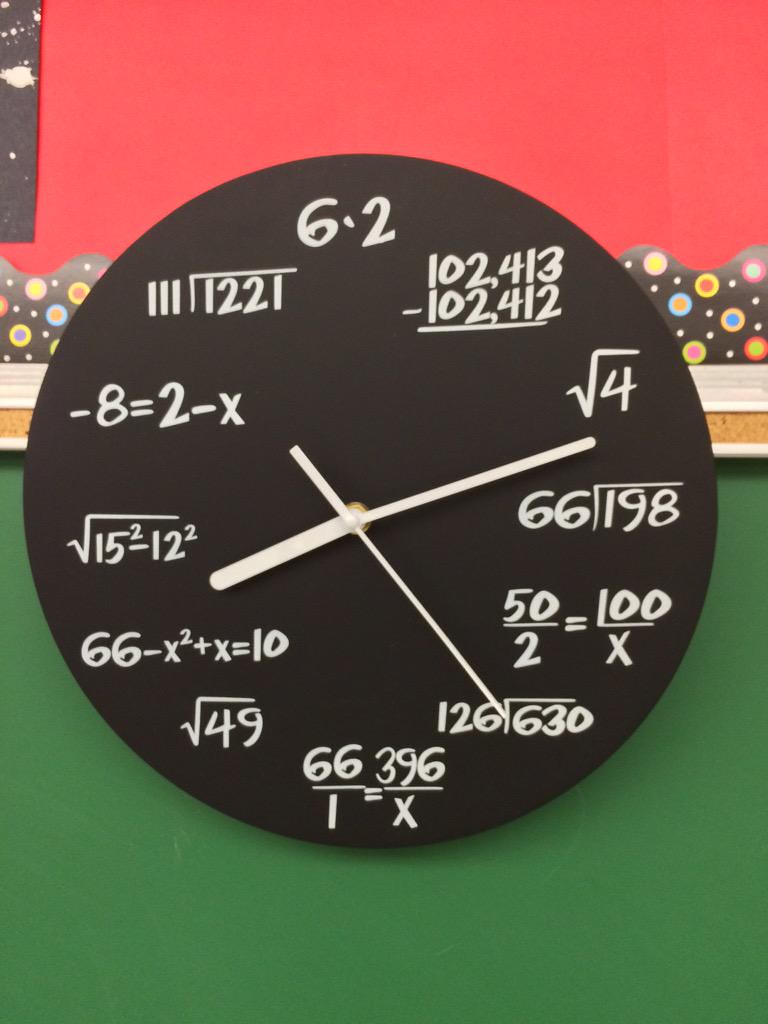This image depicts a round, black wall clock designed to resemble a chalkboard, with mathematical equations representing the hours in place of traditional numbers. Notably, 12 o'clock is displayed as "6 × 2," and 1 o'clock is represented as "102,413 - 102,412," while 2 o'clock is the "square root of 4." The clock is detailed with three white hands for the hour, minute, and second, and lacks a glass cover or frame. It's mounted on a wall with a distinct background: the upper portion is red, the lower portion is green, and along the middle section, there's a strip of white molding with a cork trim. The upper portion also features a black wallpaper trim adorned with colored polka dots just above the molding, suggesting the setting could be a playful, educational environment like a child’s classroom.